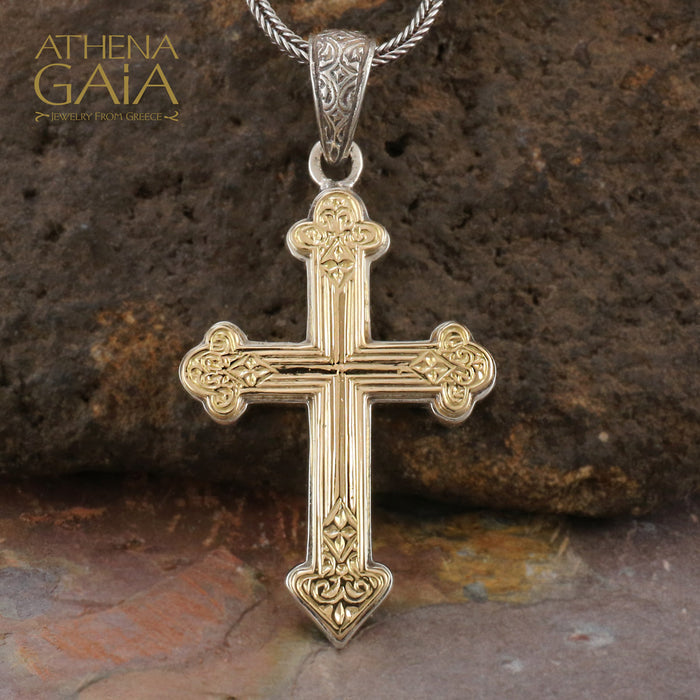This image showcases a detailed and ornate golden cross pendant hanging from a silver ring, with intricate scroll-like and gothic patterns at the ends of its arms. The cross, about five inches long, also features a touch of silver in its center. The pendant is positioned diagonally on a piece of slate, which itself rests on a rough, dark brown stone surface. In the upper left-hand corner of the photograph, the watermark "Athena Gaia" appears in a dark yellow or orange hue, accompanied by the text "Jewelry from Greece." The overall composition highlights the craftsmanship and intricate designs of the cross against a dark, textured background.